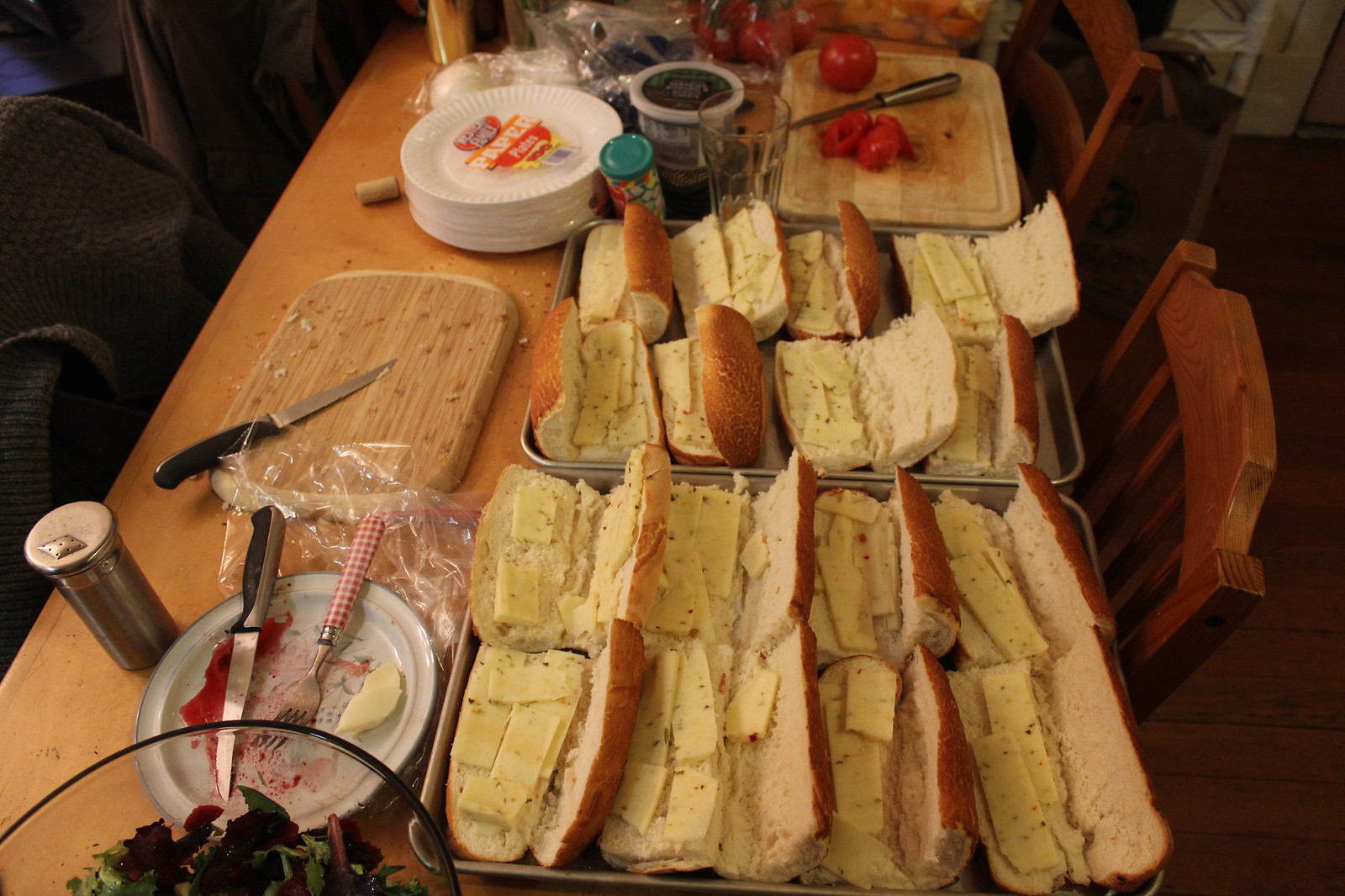An overhead view captures a long rectangular butcher block wooden table surrounded by chairs—two brown chairs on one side and a gray chair with a sweatshirt draped over it on the left. The table is laden with the makings of an extensive sandwich preparation. Two silver trays, one holding eight and the other ten split-open sub-rolls, each lined with pepper jack cheese speckled with spices, occupy the center. To the left, a scene of active kitchen use is evident: a wooden cutting board with a knife, a dirty white plate with a knife and fork, and a half-visible bowl filled with green salad. Additional elements include a stack of wrapped white paper plates in the upper left corner, another cutting board with partially sliced tomatoes, a tub potentially containing dip, and a bag of white onions in the background. The detailed setup suggests an ongoing and meticulous preparation of a large batch of sandwiches.